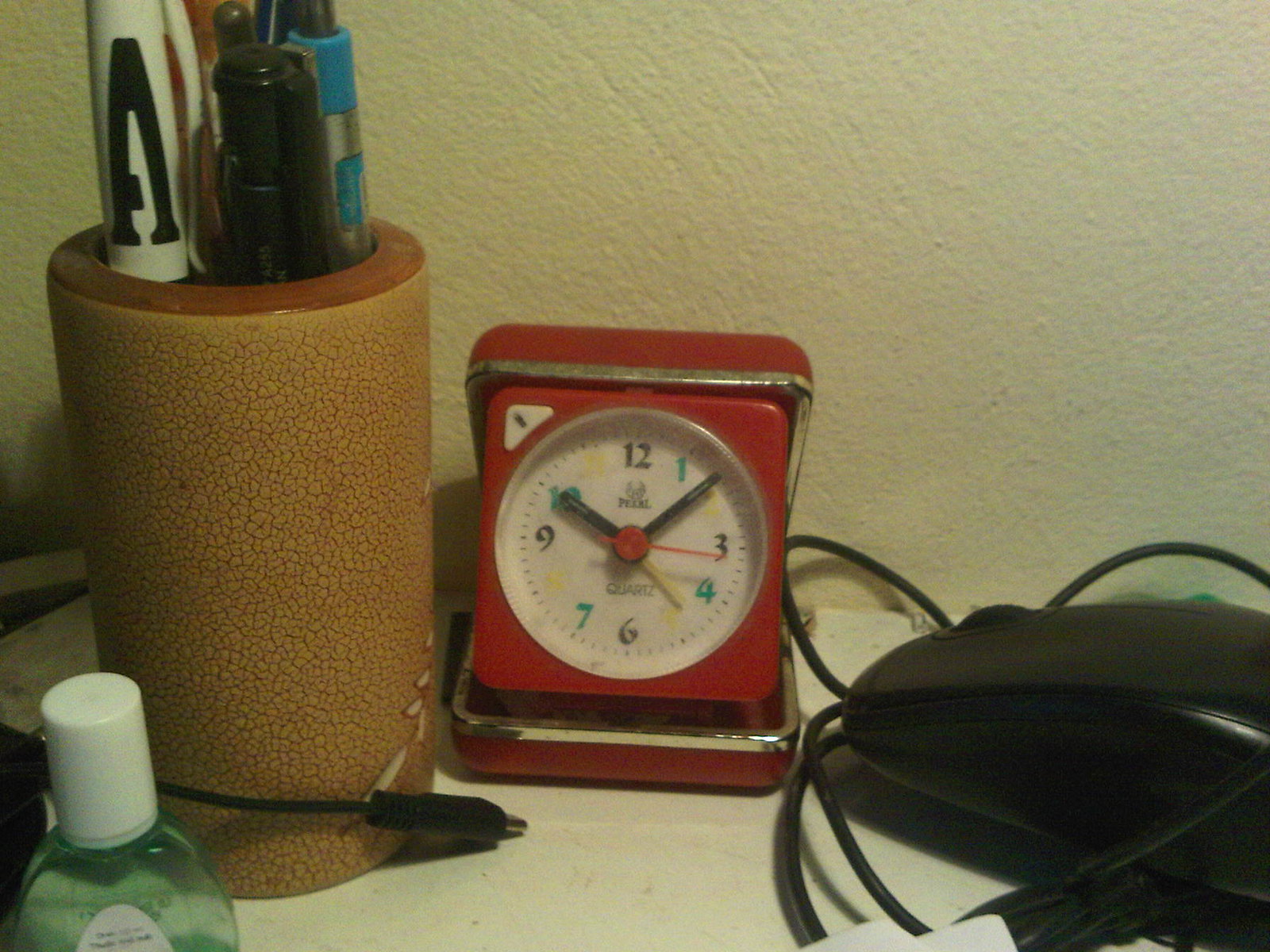A small table area is neatly arranged against a textured cream-colored plasterboard wall. The table itself is white with subtle flecks, adding a bit of character to its surface. Dominating the center of the table is a red travel clock encased in a protective red case with a silver rim. The clock features a white face, surrounded by a vibrant red border, and is covered by a clear plastic shield. The clock's hands are black, with a red second hand and a distinct yellow hand for the alarm. The numbers on the clock are color-coded: 1, 4, 7, and 10 in green; 2, 5, 8, and 11 in yellow; and 12, 3, 6, and 9 in black. The current time displayed is 10:08 and 16 seconds, with the alarm set for 10:30.

To the right of the clock, a black device, possibly a phone or a mouse, sits connected by a cable. On the left side of the table, a pencil holder made of green or brown leather-like material is wrapped with a charger. The holder contains an assortment of writing instruments, including a black pen, a silver pen with blue accents, and a white pen marked with an 'A' on its cap. In the left corner of the table, there is a bottle, likely containing hand cleaner. The bottle features a white cap, a greenish-clear liquid inside, and a partially visible white label.